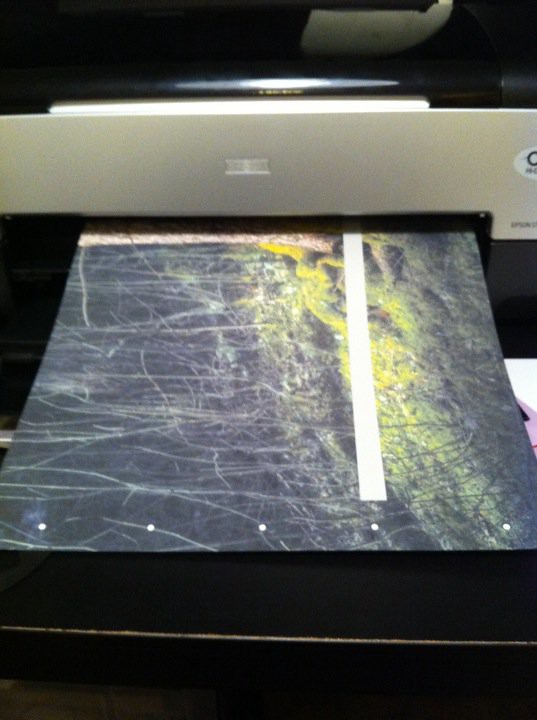The image captures a silver-colored laminator or scanner, positioned on what appears to be an office desk. To the right side of the equipment, an oval shape is partially cut off by the edge of the picture, with a black circle and black lettering visible below it. An additional level on top of the equipment features a slot from which a dark-colored picture is emerging. The picture depicts a landscape scene with branches, grass, and a few yellow flowers. A thick white rectangular box overlays the yellow flowering, while on the right side of the picture, there appears to be a larger tree extending onto a black surface. The sheet of paper being processed also shows a detailed green grassy ground with bare thorns or vines, further adding to the intricate botanical imagery. The overall presentation suggests a complex and somewhat unfinished print output.